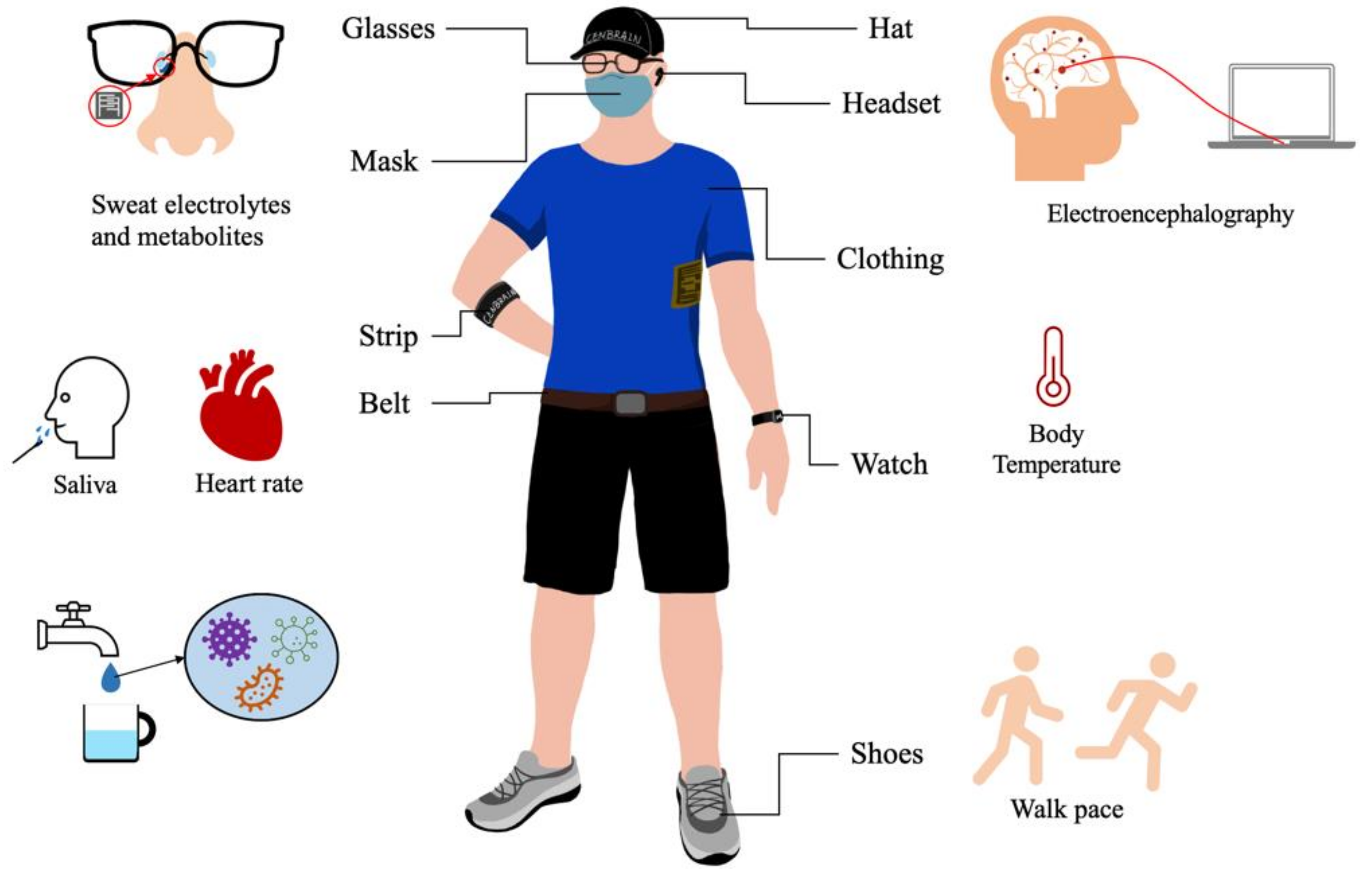The image showcases a detailed, computer-generated graphic of a man on a white background. He is depicted wearing a blue short-sleeved top, black shorts, a brown belt with a silver buckle, and gray tennis shoes. Adorning his face are black eyeglasses, and he has a black ball cap perched on his head. The man is also wearing a light blue COVID-era mask.

Surrounding the man are numerous icons and labels in black text that highlight various health-related metrics. These include a heart rate monitor, indicators of sweat, electrolytes, and metabolites, and details about his nose and glasses. There are also visuals depicting saliva, a heart, drinking water, walk pace, body temperature, and an electroencephalography (EEG) link from his brain to a laptop computer. This comprehensive graphic appears to illustrate various bodily functions and health parameters, potentially within the context of COVID-19 safety and monitoring.